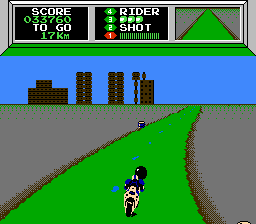This image is a detailed screenshot from a vintage-style motorcycle video game. The game's backdrop features a deep blue sky and a silhouette of block-like buildings, including four large skyscrapers—two on each side—with a smaller rectangular building and a skinny tower to the left. The central scene shows a motorcycle rider, distinguished by a black helmet and a blue shirt, riding a tan motorcycle with black wheels. The rider is navigating a green road marked with green hash lines, against a mid-gray to dark gray outer road boundary. The interface includes a gray rectangle at the top displaying the score "033760" in green, the distance to go "17KM" in white, and various game status indicators like the rider's remaining lives and shots left. The simple, yet nostalgic graphics suggest a gameplay style reminiscent of the 1990s.